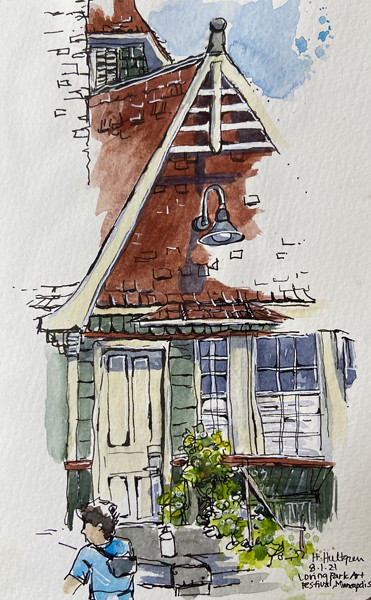The artwork depicts a detailed drawing featured on a rectangular sheet of paper, oriented in a portrait view against a light gray background. The focal point of the illustration is the front façade of a house. The house boasts a warm brown roof and is adorned with green siding. Prominent white columns frame the windows and a pristine white door stands at the center, offering a welcoming entrance. 

Affixed to the house is a modest gray front porch, bordered by vibrant plants in hues of light green and yellow, adding a touch of natural beauty to the scene. Adding human interest to the drawing, the bottom left corner captures the back of a man. His grayish hair hints at maturity, and he is casually dressed in a blue t-shirt. A gray fanny pack is slung across his shoulder, suggesting preparedness and simplicity. The composition successfully combines architectural detail with an element of everyday life, providing a sense of comfort and familiarity.